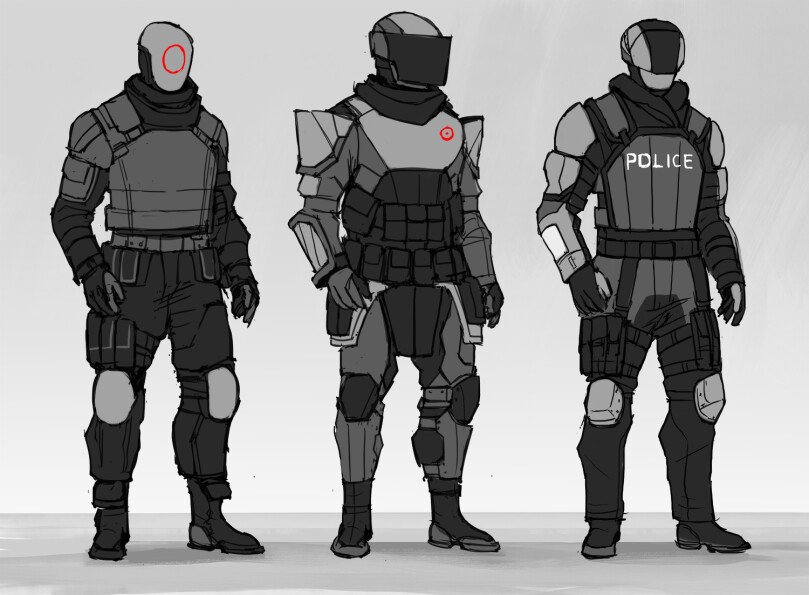The image appears to be concept art, possibly for a comic or an anime, featuring three characters dressed in tactical police uniforms. The figures are adorned in black and grey attire, with heavy gear including helmets, shin guards, bulletproof vests, and various pouches likely for carrying weapons. Each character has unique features: the one on the left wears a helmet marked with a red circle; the middle figure sports spiky shoulder pads, a black visor, and a red dot on his chest; and the far right character, who has "POLICE" written in white font on his chest, completes the trio. The overall palette of the artwork consists of black, grey, white, and touches of red, suggesting a gritty, possibly futuristic or sci-fi theme.